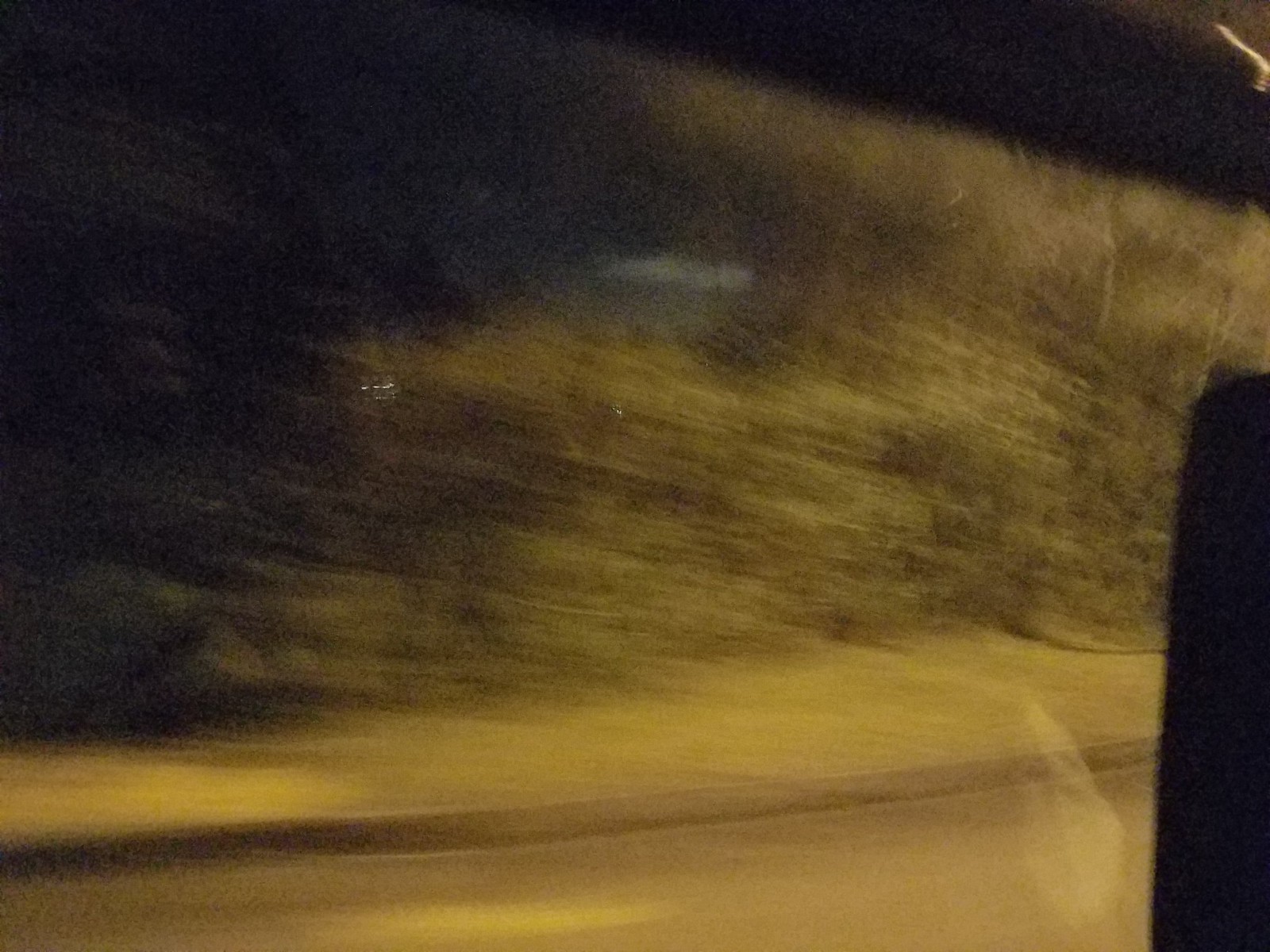The photograph is taken from inside a moving vehicle, offering a view through the window. The scene outside presents a blur of motion with a cluster of green bushes swept towards the left, indicating the direction of the vehicle's travel. The foliage transitions from a vibrant green to a lighter shade, ultimately darkening to nearly black towards the edges. Below the bushes, there's a small patch of grass, barely noticeable, leading into a curving gray path that morphs into a road.

Amidst the shadowy dense bushes, an eerie visage seems to emerge—marked by long, horizontal white eyes and a faintly perceptible mouth, which creates an unsettling, almost spectral effect as if a light is reflecting back ominously. This subtle, haunting face-like figure adds a mysterious element to the otherwise everyday roadside scenery.